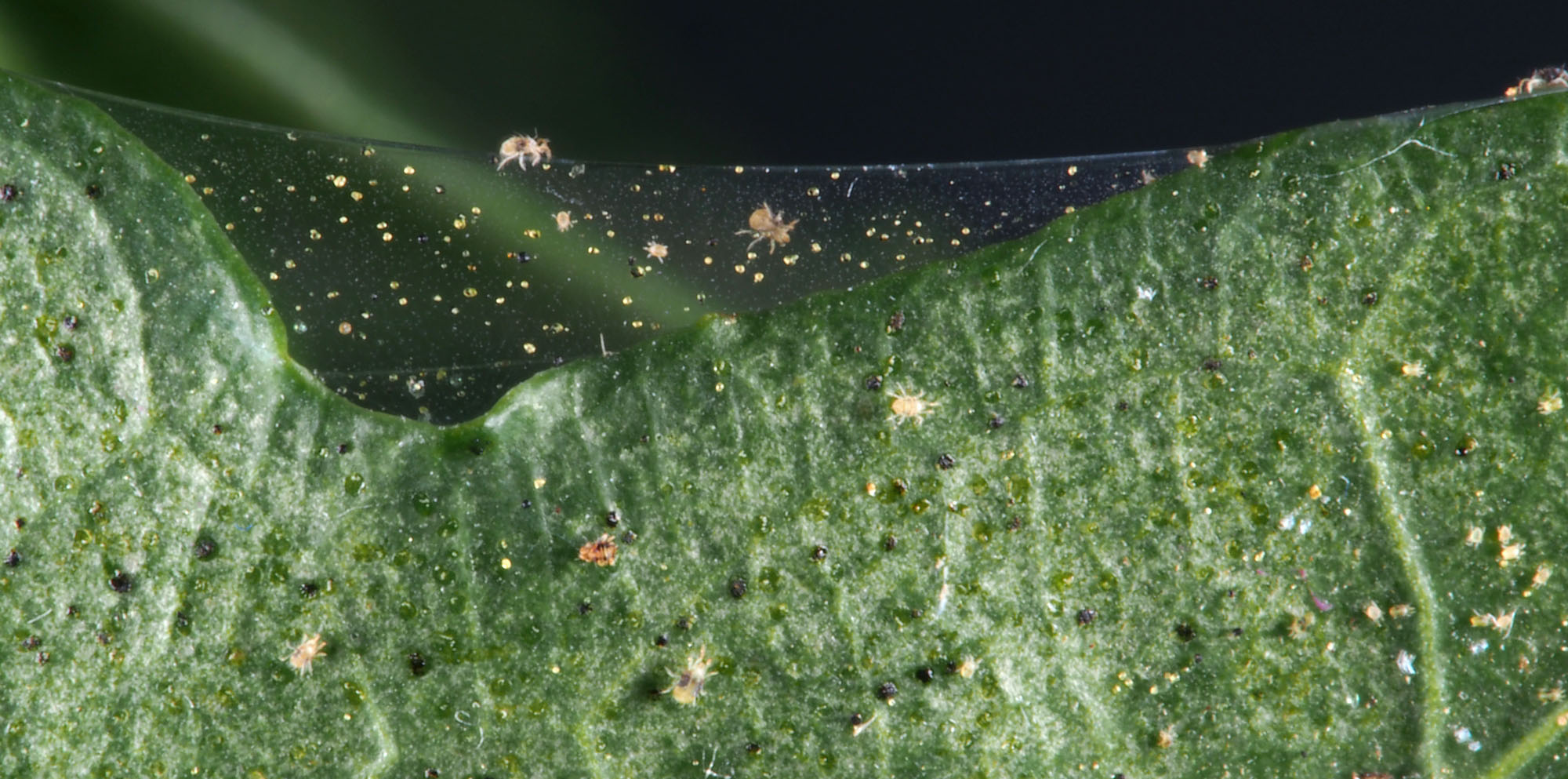A close-up image captures the eerie presence of a dense spider mite web enveloping a green plant, reminiscent of lettuce. The thick, hasty weave of the web is cluttered with countless spider mites, distinguished by their brown and white hues, indicating various stages of growth. Amidst the teeming mites, clusters of eggs are visible, varying in color from yellow to brown and black. Known pests in agricultural settings, these spider mites pose a significant threat as they infest and feed on crops like corn. The overall scene is unsettling, with the plant suffocated under a network of webbing and a swarm of crawling mites and eggs.